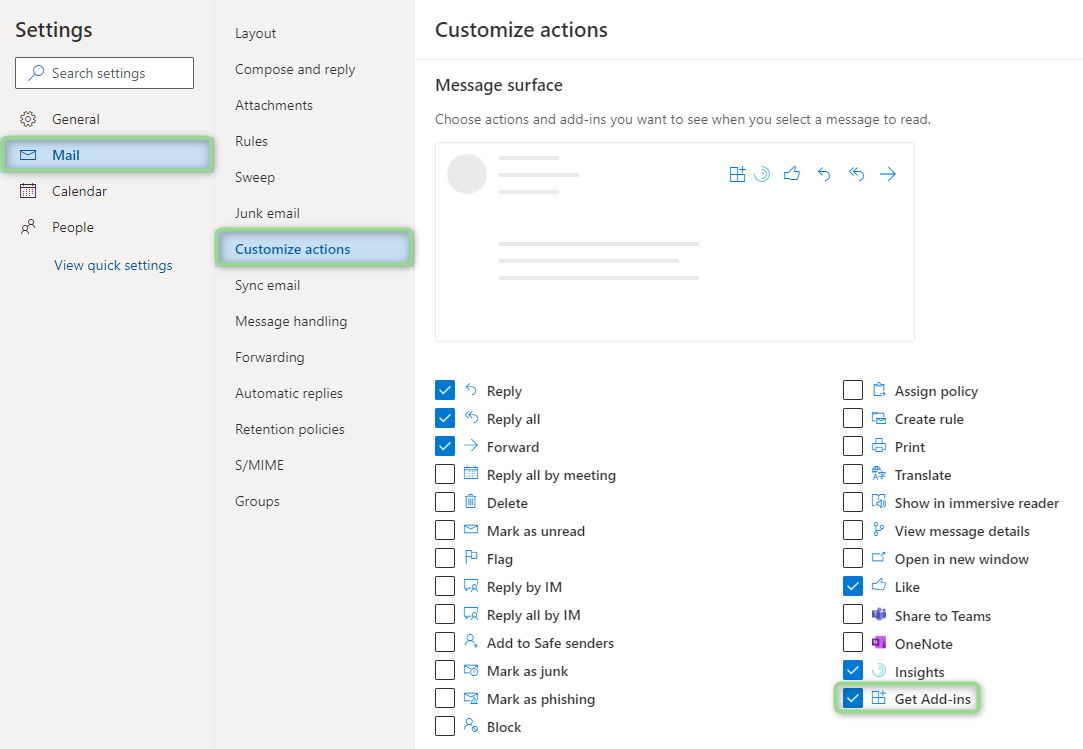Caption:
"The image depicts a detailed settings menu within an email client. The interface is enclosed in a gray rectangle. On the left side, there is a search bar above various categories: 'General' with a cog icon, 'Mail' with a mail icon, 'Calendar,' and 'People'. The 'Mail' category is actively selected, indicated by a green-outlined blue bar. 

At the bottom of this sidebar, there is an option 'View Quick Settings' in blue text. Adjacent to this sidebar, on the right, there is a more detailed menu, listing options from top to bottom: 'Layout,' 'Compose and Reply,' 'Attachments,' 'Rules,' 'Sweep,' 'Junk Email,' 'Customize Actions' (highlighted in blue with a green outline), 'Sync Email,' 'Message Handling,' 'Forwarding,' 'Automatic Replies,' 'Retention Policies,' 'S/MIME,' and 'Groups.'

Under the 'Customize Actions' section, it reveals various checkboxes for actions such as: 'Reply,' 'Reply all,' 'Forward' (all checked), and additional options like 'Reply all by meeting,' 'Delete,' 'Mark as unread,' 'Flag,' 'Reply by IM,' 'Reply all by IM,' 'Add to safe senders,' 'Mark as junk,' 'Mark as phishing,' 'Block,' 'Assign policy,' 'Create rule,' 'Print,' 'Translate,' 'Show in immersive reader,' 'View message details,' 'Open in new window,' and a few more. Several of these options, including 'Share to Teams,' 'OneNote,' 'Insight,' and 'Get Add-ins,' are selected, with 'Get Add-ins' highlighted in a green-outlined box.

This comprehensive settings menu allows users to customize their email experience extensively."